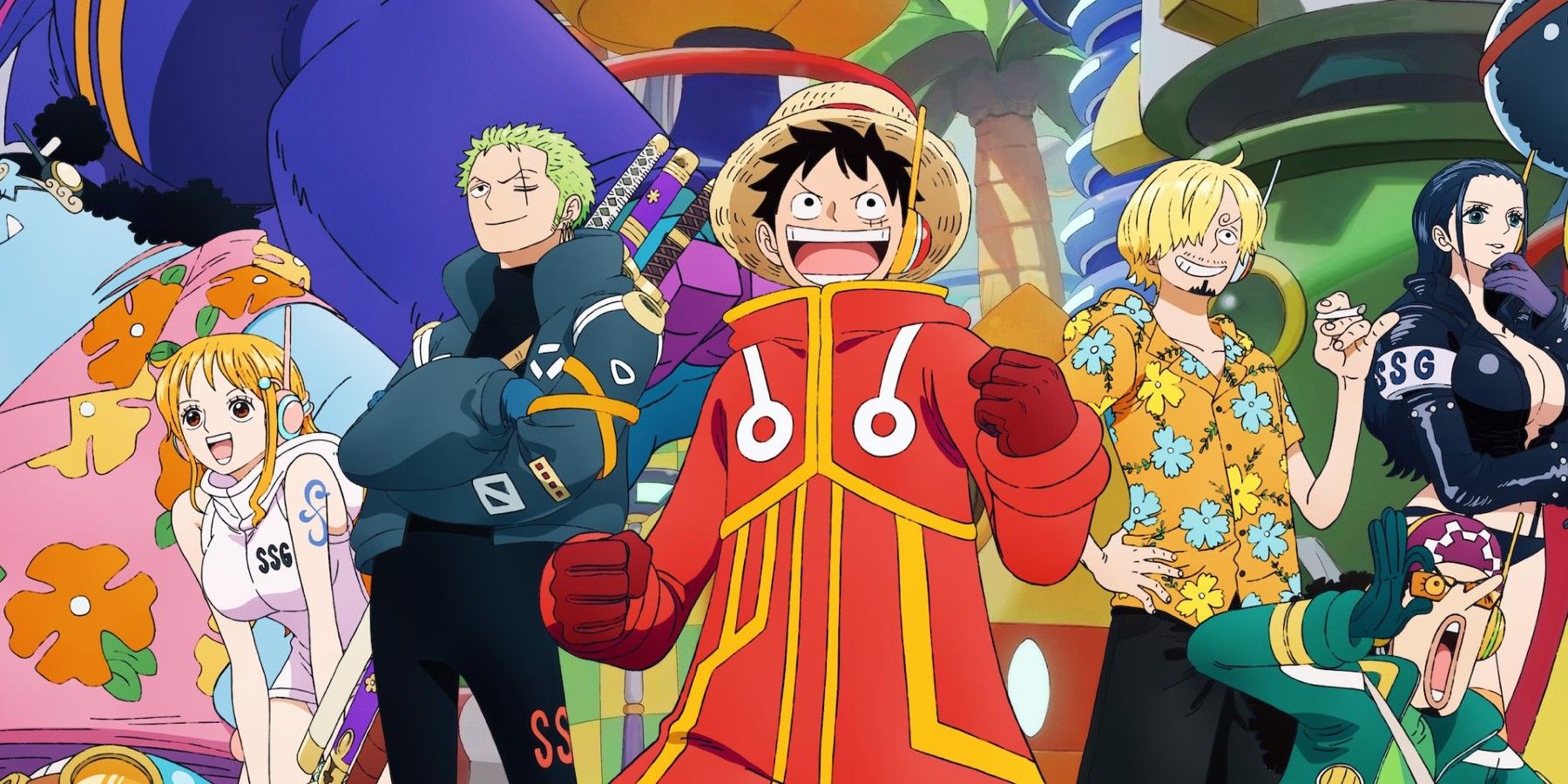This vibrant and colorful image from the anime One Piece features a central figure, Monkey D. Luffy, recognizable by his signature broad-brimmed straw hat with a red band. Luffy is depicted with a wide-open mouth and excited expression, wearing an eye-catching outfit that includes a yellow-white jacket with red gloves and white detailing.

To Luffy’s left, we see Roronoa Zoro, identifiable by a prominent scar over his left eye and his three swords slung over his back. Zoro is dressed in a puffy green coat and navy pants featuring the letters "SS" on the left leg. Standing next to him is Nami, who has orange hair, wears headphones, and dons a white, skin-tight bodysuit with "SSG" emblazoned on the left side of her chest.

On Luffy’s right, the blond-haired Sanji wears an orange Hawaiian shirt, black pants, and holds a cigarette with a big smile. Near Sanji, Usopp, crouching in the lower right-hand corner, is characterized by his long nose and a purple bandana with white checks in a star pattern. He is depicted yelling with a cupped hand near his mouth, dressed in a green shirt, teal jacket, and dark green gloves.

Behind Usopp, Nico Robin stands pensively, her jacket unzipped to reveal a dark purple bikini. She has dark purple hair and the "SSG" insignia on her right shoulder. The backdrop showcases vibrant and stylized elements such as a pineapple tree, roundish buildings, and a large Hawaiian-themed sheet with floral patterns, adding to the lively atmosphere of the image. Overall, the scene captures the dynamic and diverse personalities of the One Piece crew.